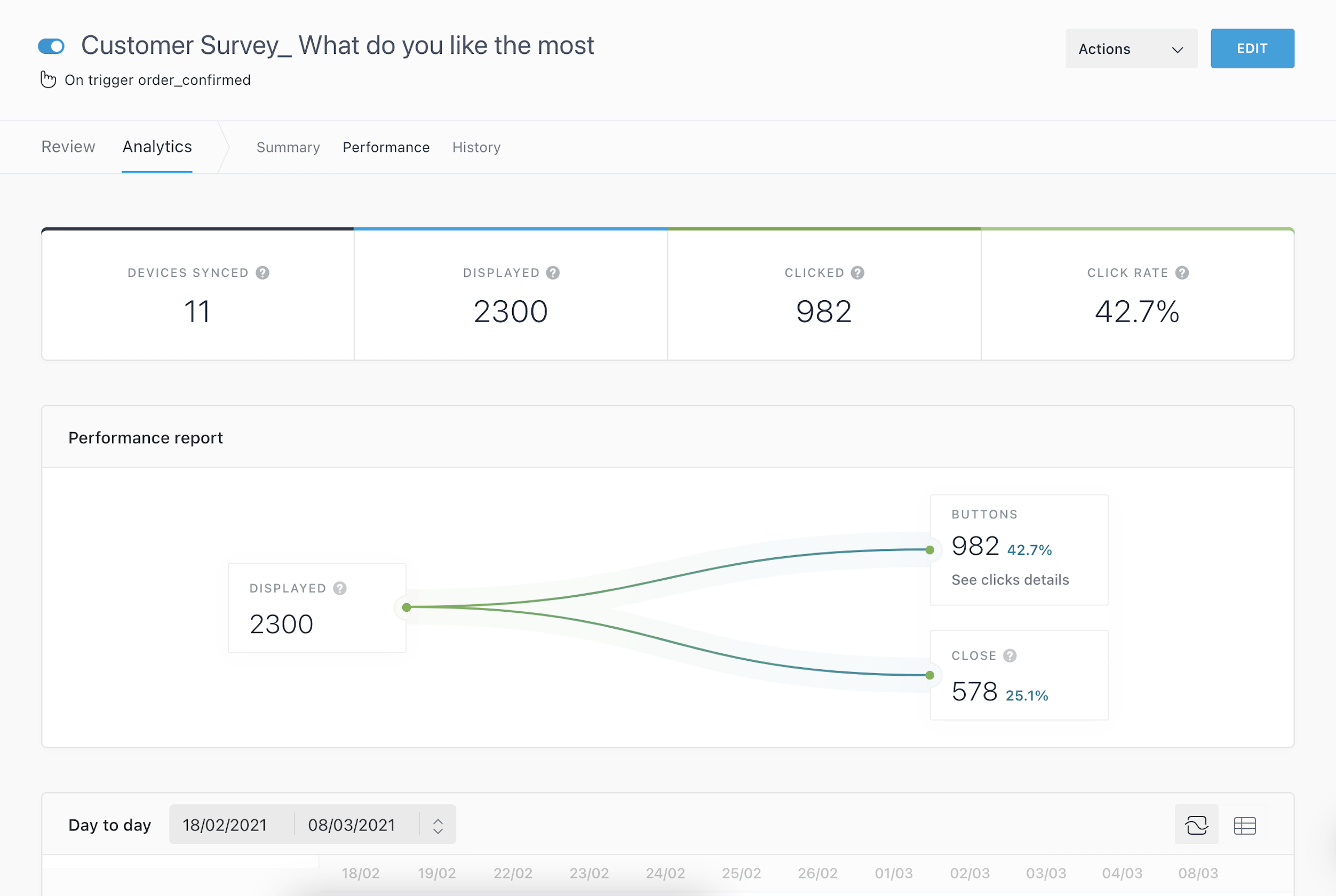The image depicts a detailed screenshot of a customer survey webpage. At the top left corner, the heading reads "Customer Survey" and directly beneath it, the prompt "What do you like the most?" appears, followed by the trigger text "Order Confirmed." A small icon of a finger points upwards towards this description. Adjacent to this, a toggle switch is visible, currently in the 'on' position. 

In the upper right section, there is a drop-down menu labeled "Actions," and next to it, a conspicuous blue button marked "Edit." The top toolbar spans options such as Review, Analytics, Summary, Performance, and History, with 'Analytics' highlighted by a blue underline, indicating the active section displayed on the main body of the page.

Dominating the central part of the screen is a performance report titled "Performance Report," timed at 23:00. Two diverging lines originate from the same point—one ascending and the other descending. The upward line, labeled "Buttons 982, 42.7%," shows an increasing trend, while the downward line, which stops next to a box labeled "Close 878, 25.1%," indicates a decreasing trend.

Additional metrics shown include "Devices Synced: 11," "Displayed at: 23:00," "Clicked: 982," and "Click Rate: 42.7%." This detailed screenshot appears to be part of an analytics dashboard for a website, although the specific nature of the tracked data remains unclear.